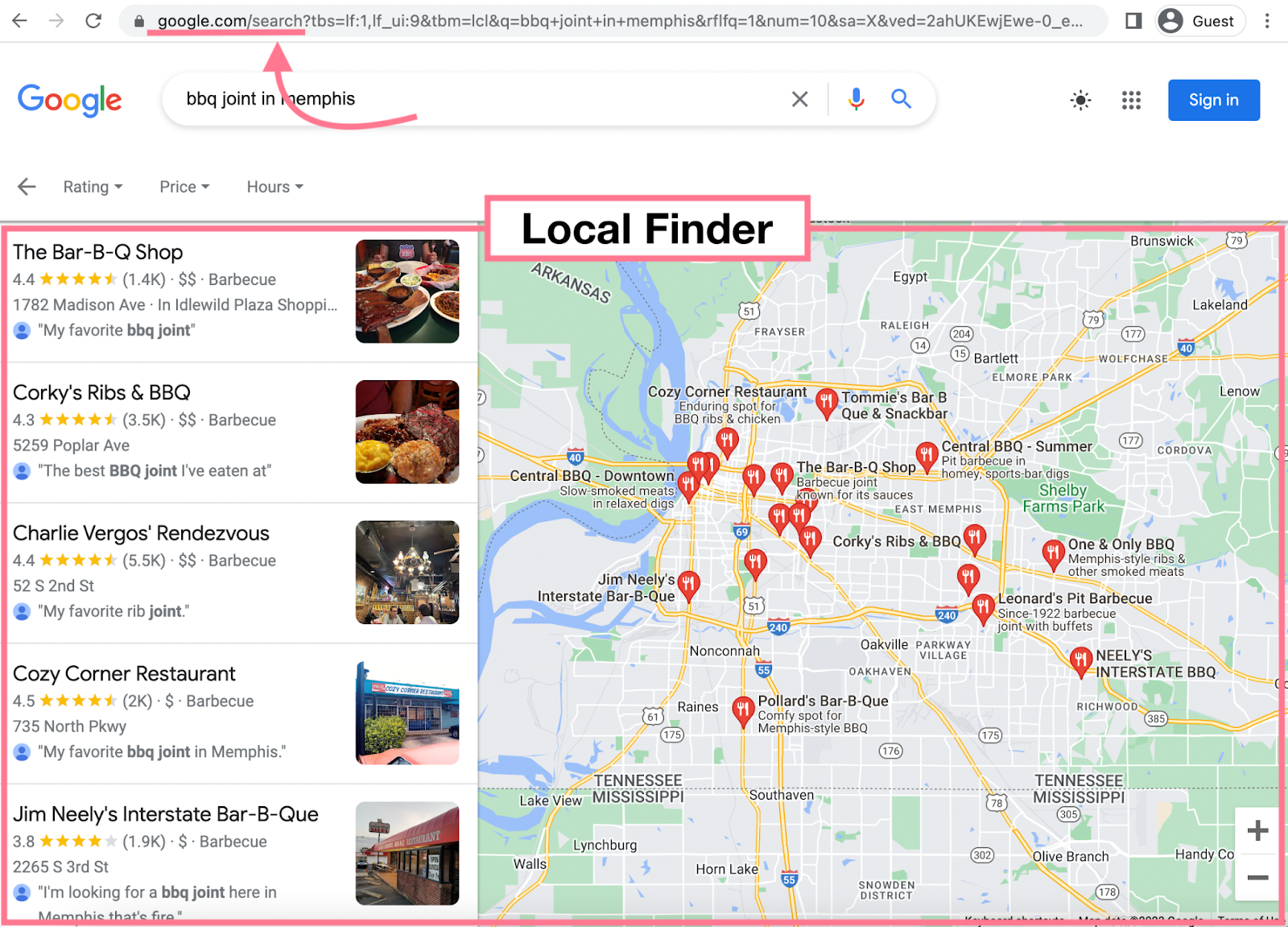The image is a detailed screenshot of a Google search results page for "barbecue joint in Memphis." At the top of the image, a red arrow points to the browser's address bar, which displays "google.com/search," and the text is underlined in red for emphasis. Below the address bar, the familiar Google logo is prominently displayed next to the search bar, which shows "barbecue joint in Memphis" as the search query. The search bar also includes icons for a microphone and magnifying glass. To the side, there are additional interface elements such as a blue "Sign In" button and vertical ellipsis indicating more options.

Beneath the search bar, there are various interactive features including ratings, prices, and hours of operation, each indicated with corresponding arrow icons. These elements are organized neatly, guiding the user to explore more detailed information.

A red box frames the main search results and an adjacent map. The term "Local Finder" is highlighted above the map, also enclosed within a red box. The search results include a list of well-known barbecue restaurants in Memphis: The Bar-B-Q Shop, Corky's Ribs and Barbecue, Charlie Vergos' Rendezvous, Cozy Corner Restaurant, and Jim Neely's Interstate Bar-B-Q. Each entry appears with its name and rating.

On the right side of the image, a map of the Memphis area is displayed with pins indicating the locations of the mentioned barbecue restaurants. The map clearly labels the Tennessee-Mississippi border, suggesting that the area in focus lies along this boundary. The layout is typical for a Google search results page, providing both a list view and a geographical view to facilitate easy navigation and selection of dining options.